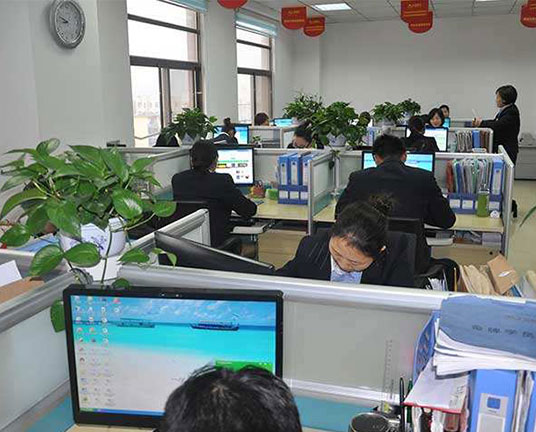In an office setting with white walls and a white tiled ceiling, two windows are situated near the top left corner of the image, accompanied by a circular clock mounted on the white wall. Red banners hanging from the ceiling add a splash of color. Rows of cubicles dominate the space, each separated by glass dividers and furnished with plain beechwood desks. Potted green plants adorn the tops of the cubicles. Workers, dressed in black suits as part of their traditional business attire, occupy the office, each diligently focused on their computer monitors displaying Windows XP desktops. In the foreground, the back of a person's head is visible as they work at their desk. A lady in a black suit stands in front of another woman seated at a computer. Scattered throughout the cubicles are file folders, books, and binders, contributing to the busy atmosphere. The colors in the image include shades of gray, silver, red, green, blue, light blue, green, and pink, capturing the professional and industrious environment of the office.